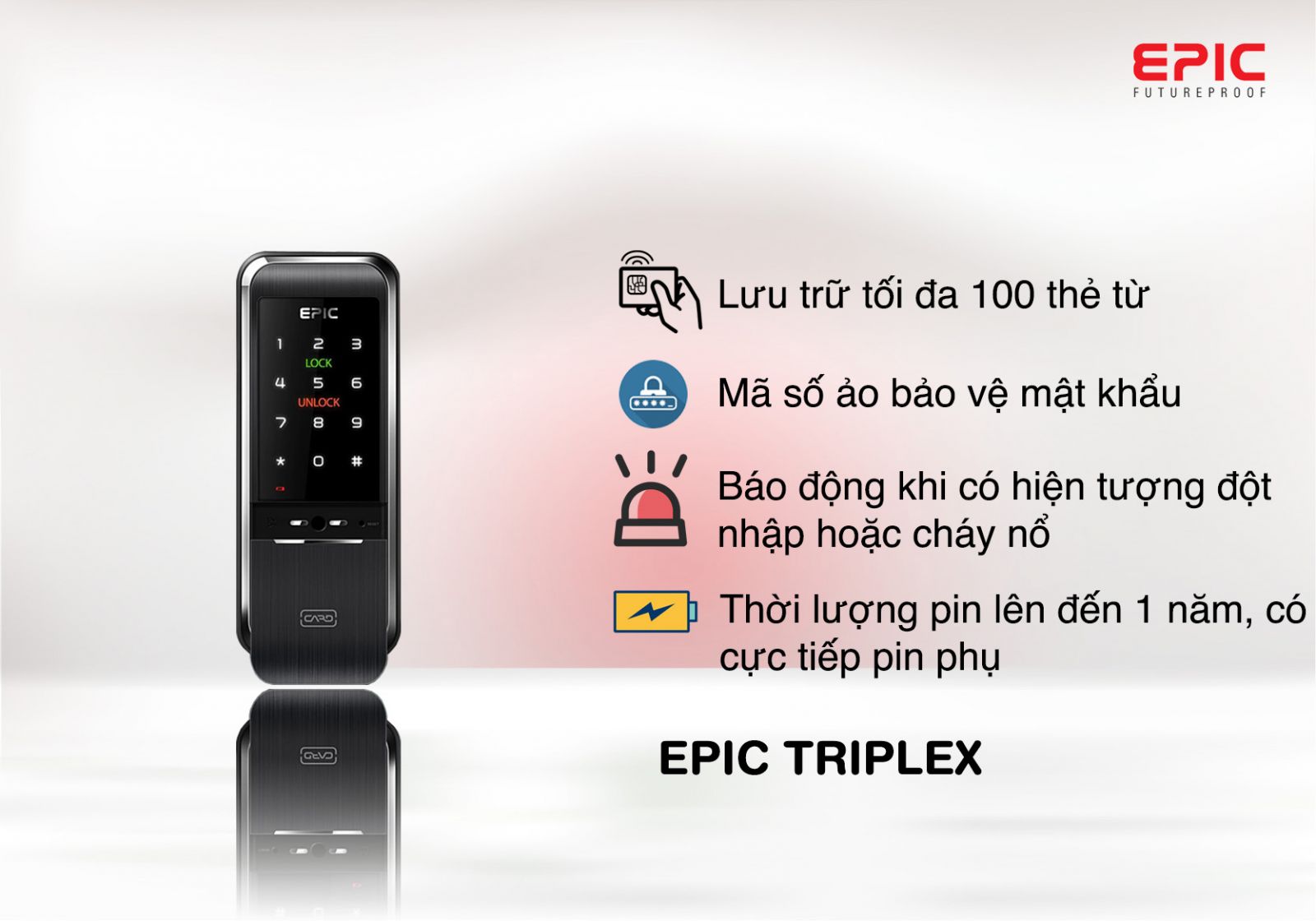The image is an advertisement for a black, tall rectangular device, which might be a phone or a security device due to its number pad and the presence of "lock" and "unlock" buttons. The number pad features the digits 0-9 along with a star (*) and pound (#) sign. The device has a silver chrome trim on the sides and is set against a soft-focused, mirrored background with a gray-to-red gradient. At the top right corner, in red and black lettering, the brand name "Epic Future Proof" is prominently displayed. Alongside the device, there are four icons to the right, each representing different features: a hand holding a credit card symbolizing wireless payment, a blue circle with a lock, a red siren, and a yellow battery with a lightning bolt indicating charge status. The ad also features the text "Epic Triplex" at the bottom. The remaining information is in a foreign language, adding to the intrigue of the product.